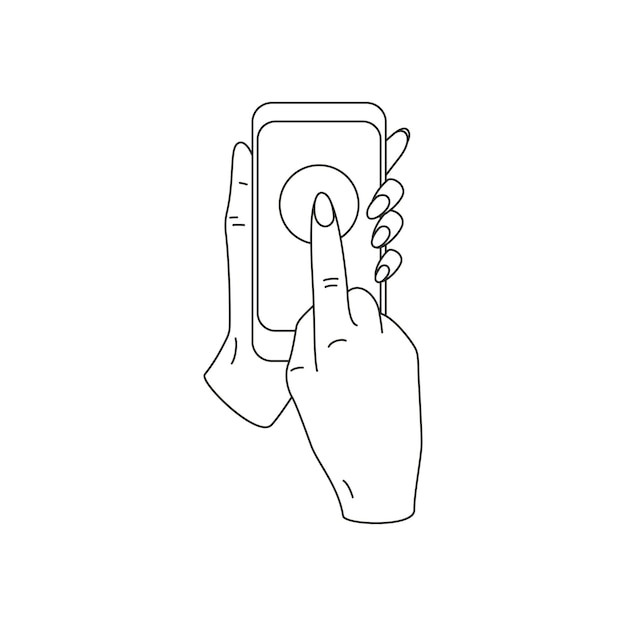In the black and white line drawing, against a stark white background, two hands are depicted engaging with a rectangular object that resembles a touch screen cell phone. The left hand, with neatly manicured and elongated fingernails, grasps the device with its thumb facing up and palm open. The rectangular object also contains a smaller, similarly shaped rectangle within it, and inside this secondary rectangle is a prominent circle. The right hand, only partially visible as it's mostly closed, extends its middle finger to press the central circular button. The scene is rendered in clean black outlines, with sparse detailing to indicate knuckles and nails on both hands.